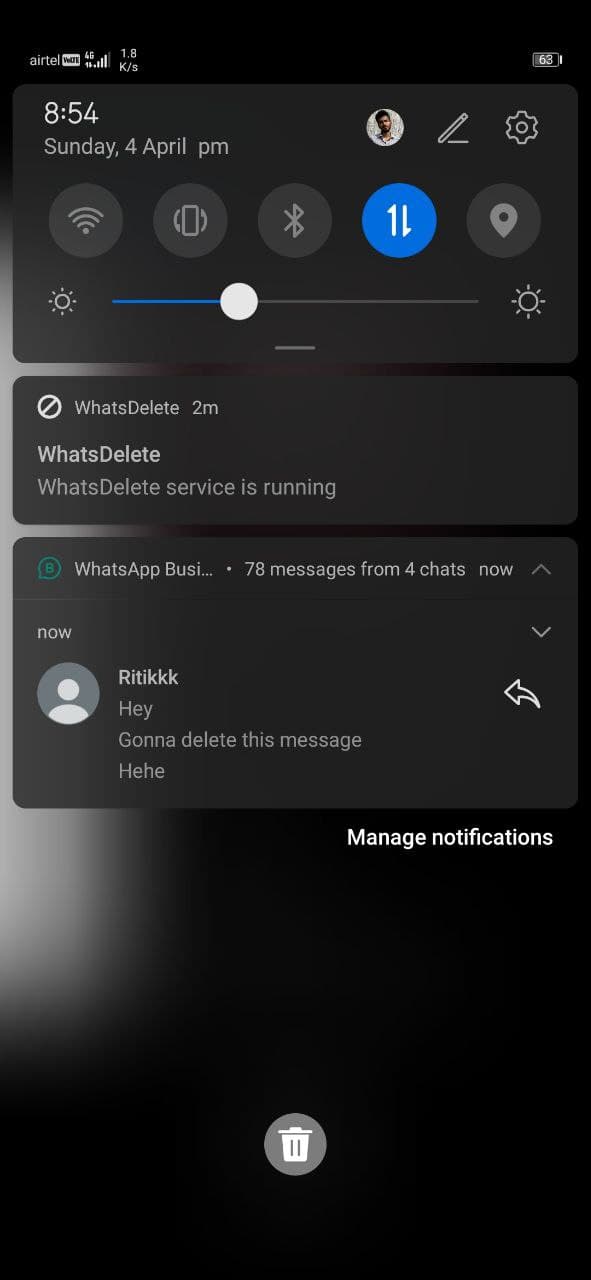This image shows the home screen of a mobile phone, specifically focusing on the settings area. The interface features three distinct rectangular sections, here referred to as bubbles, each with a predominantly light to dark grey gradient background. 

The first bubble displays information and icons in a row. It has a black background and shows the time and date as "8:54 PM, Sunday, April 4." Below this, there are five icons arranged horizontally indicating cell phone signal, portrait orientation lock, Bluetooth connectivity, data usage (up and down arrows), and location services. Additionally, there is a brightness adjustment slider beneath these icons, which gradually transitions from darker on the left to lighter on the right. Topping this section is a small picture avatar, presumably of the user, alongside a gear button for accessing further settings.

The second bubble appears to be a notification panel or quick access feature. The primary content of this bubble is not entirely clear, possibly due to a recognition error in the voice caption. The text here ambiguously states "What's delete at 2 PM. What's delete? What's delete? Services running."

The third bubble pertains to "WhatsApp Business," indicating an active session or notification related to the app. Also present within the interface are a return icon on the right side and options to manage notifications or delete items, with the trash icon located at the bottom center of the screen.